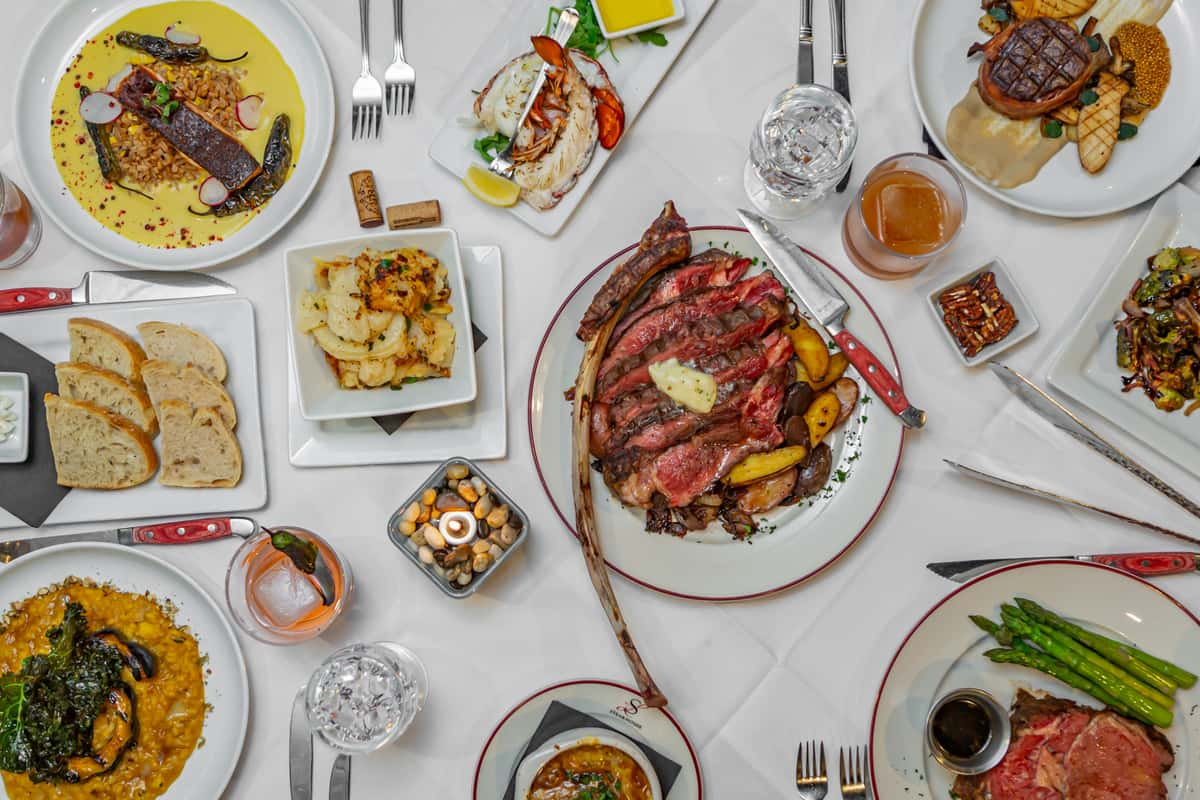This photograph captures a bird's-eye view of a beautifully arranged circular table covered with a white tablecloth, laden with a myriad of dishes and beverages. At the center, the focal point is a large plate showcasing a tomahawk steak, which appears undercooked with a red interior and brown exterior, and it is accompanied by potatoes and mushrooms, topped with a piece of butter and a carving knife. Surrounding this central dish, the table boasts a variety of culinary delights: plates of asparagus, risotto, salmon steak, lobster tails with a butter dipping sauce, and grilled chicken with gravy. Small bowls of nuts and snacks are interspersed among the dishes, alongside soups and fresh bread. The place settings include various utensils, neatly arranged with knives, forks, and spoons, while an assortment of drinks—water, juices, and possibly other beverages—are carefully placed in glasses around the table. Adding to the elegant presentation, there's a decorative centerpiece featuring a glass container filled with rocks, pebbles, and a candle. The overall setup exudes a formal dining ambiance, meticulously designed for communal enjoyment.